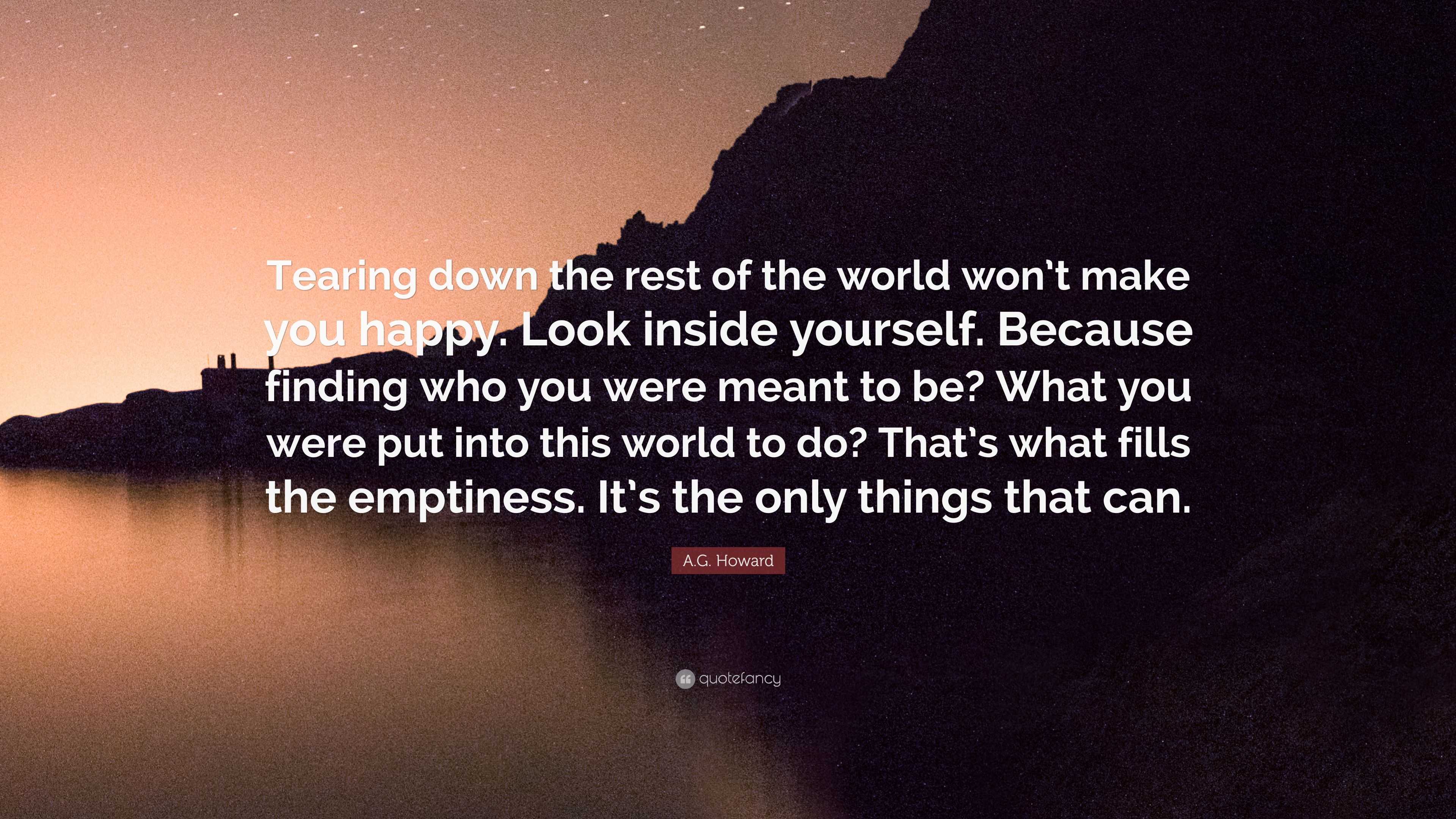The image depicts an inspirational quote set against a serene lakeside scene at dusk. In the foreground, the clear, orange-tinged water reflects the fading light of the setting sun. To the left, on the distant shoreline, a solitary building stands against a backdrop of descending, shadow-covered mountains that stretch from the upper right towards the middle left of the image, their peaks rendered almost black by the encroaching darkness. Above, the sky transitions from pale orange to deeper hues, dotted with emerging stars. At the center of the image, white text reads: "Tearing down the rest of the world won't make you happy. Look inside yourself because finding who you were meant to be, what you were put into this world to do, that's what fills the emptiness. It's the only thing that can." Below the quote, in a small brownish rectangle, the author A.G. Howard is credited, accompanied by the Quote Fancy logo.